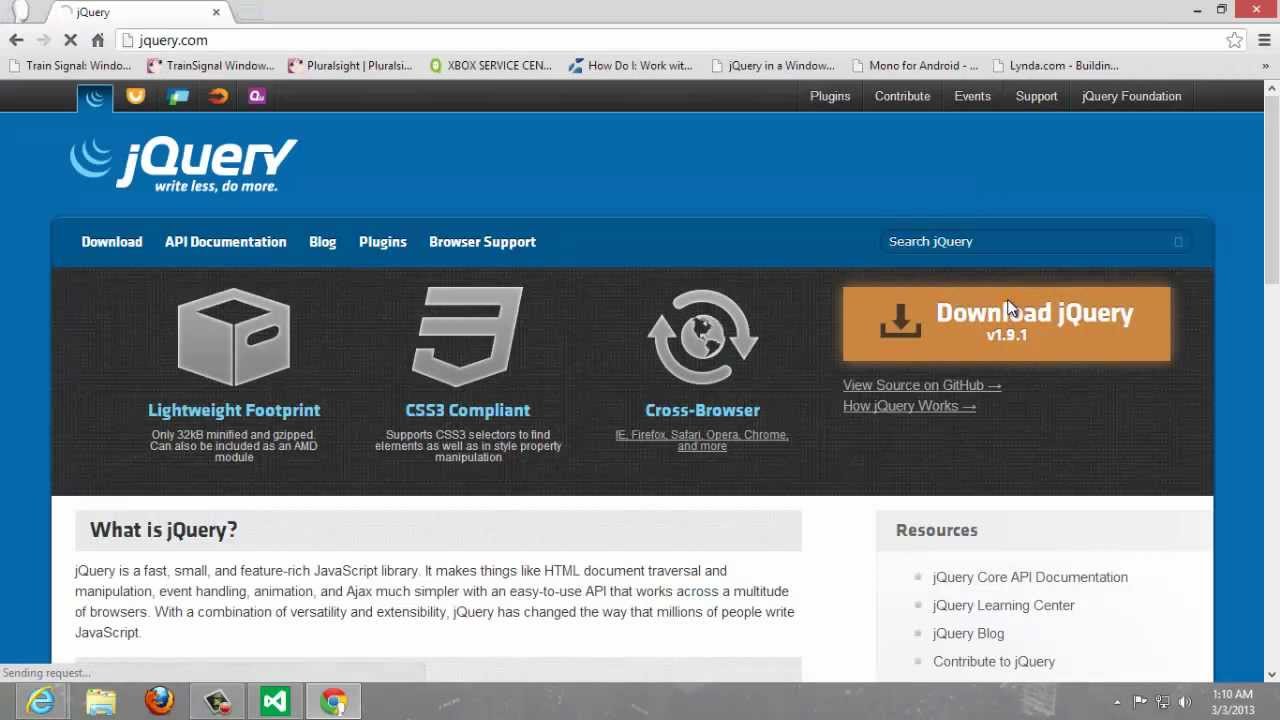The image displays a webpage from the jQuery website, showcasing the tagline "Write less, do more." At the top, the company’s logo resembles three crescent moons of varying sizes. There is a navigational tab bar that includes options for "Download," "API Documentation," "Blog," "Plugins," and "Browser Support," with a search box for querying the site positioned to the right.

Directly beneath the navigation bar are several highlighted features of jQuery: "Lightweight Footprint," "CSS3 Compliant," and "Cross-Browser Support." Each feature is accompanied by a relevant icon. The "Lightweight Footprint" is represented by an icon resembling a carry box with hand slots, "CSS3 Compliant" is denoted by a chevron-like symbol, and "Cross-Browser Support" is illustrated by a globe with arrows circling it clockwise.

To the right of these features is a prominent "Download jQuery" button, with the cursor hovering over it. Below this, the text explains, "What is jQuery?" It describes jQuery as a fast, small, and feature-rich JavaScript library that simplifies HTML document traversal, manipulation, event handling, animation, and AJAX with a user-friendly API compatible across numerous browsers. The description underscores jQuery's versatility and extensibility, emphasizing its transformative impact on JavaScript development for millions of users.

On the right side of the page, there is a resource box titled "jQuery Core Resources" which includes bullet points linking to "API Documentation," "Learning Center," "Blog," and "Contribute to jQuery."